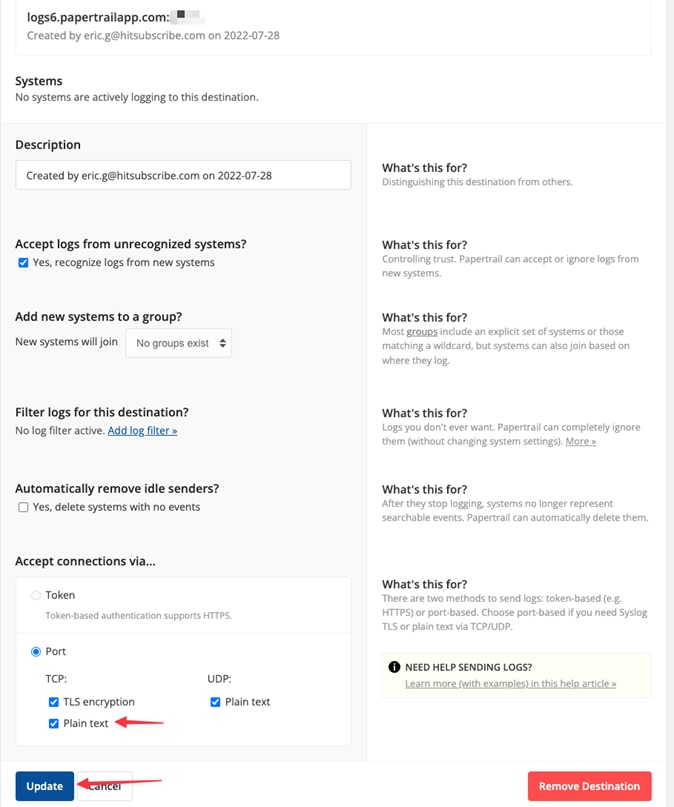The image showcases a settings page on the website "log6.papertrailapp.com". At the top left-hand corner, the website URL is clearly displayed. Adjacent to it is some information that appears to be blurred out. Beneath this, there is a line indicating that the content was created by Eric G. with the email address at hit subscribe.com, and it was created on the date 2022-07-28.

Further down, there is a notification stating that no systems are actively logging to this destination, though the word 'destination' seems to be truncated with an extra 'T' at the end. Below this notification is a box with a light gray background containing a description. Within this box, it reiterates that the entry was created by Eric, followed by the .com date.

At the bottom of this section, there is an option labeled "Accept logs from unrecognized systems," which has been checked. Below this, there is another checkbox labeled "Add new systems to a group," alongside several options including "Filter logs for the destination," "Automatically remove idle senders," and "Accept connections via," which is followed by a white box labeled "token port."
 
Additionally, there are areas with checkboxes, and there are two red arrows pointing to specific options: one directs attention towards "plain text," while the other points to "update." On the right-hand side, there is a heading "What's this for?" followed by detailed information pertaining to each question listed.

At the bottom of the image, there is a red rectangle button labeled "Remove Destination."

This detailed description not only clarifies the contents of the image but also provides insights into the functionalities and settings depicted on the page.